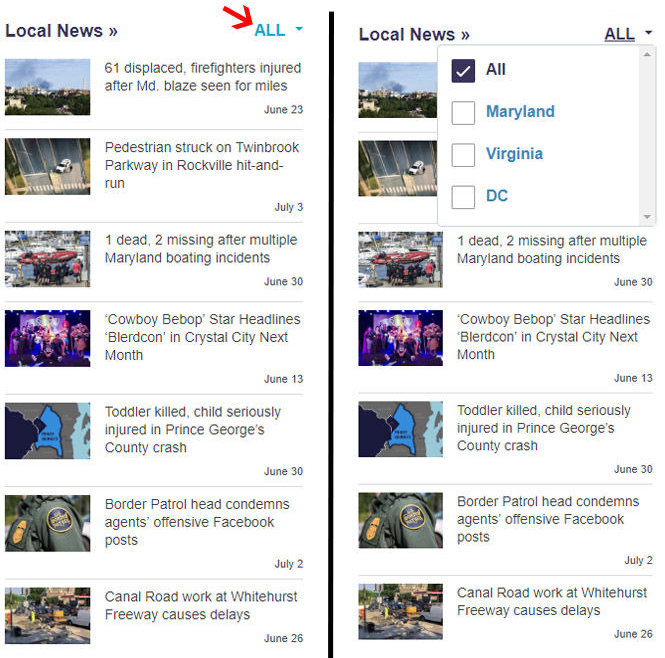The image is divided into two sections by a thin black line running vertically down the center. On the left page, the title "Local News" is prominently displayed followed by two small right-pointing arrows. On the right page, the word "ALL" is written in blue capital letters, with a bold red arrow pointing towards it. Below, there are seven distinct news stories, each accompanied by an image and a date. The headlines are dated as follows: June 23rd, July 3rd, June 30th, June 13th, June 30th again, July 2nd, and June 26th.

On the right half of the page, at the top, the title "Local News" reappears, this time in bold print and followed by the two right-pointing arrows. Below this, "ALL" is written in black print with a drop-down menu displaying options for "ALL," "Maryland," "Virginia," and "D.C." The option "ALL" is selected. The same seven stories are listed below, each with their respective dates and images displayed alongside them.